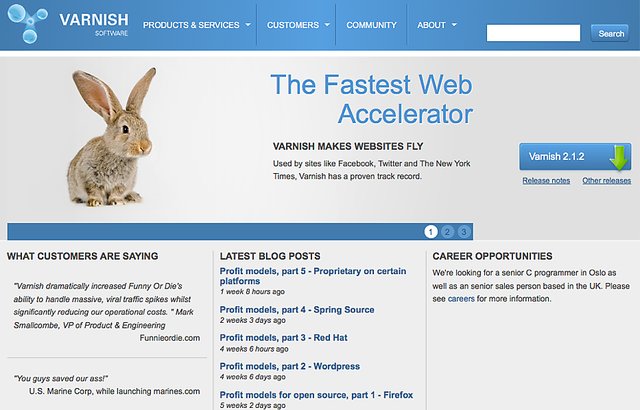In the image, a structured web layout appears as follows:

At the top, there is a blue rectangle serving as a banner, prominently featuring a light blue logo on the left-hand side. This logo consists of light blue circles interconnected by darker blue lines, illustrating a network or system. Following the logo, the word 'Varnish' is displayed, though an additional word beneath it remains illegible.

Beneath this banner, the navigation menu is laid out with titles and dropdown indicators: 'Products and Services' is followed by a downward arrow, indicating further options. Adjacent entries include 'Customers' with an arrow pointing downwards, 'Community', and 'About', also with a downward arrow.

To the right side of this horizontal menu, there's a functional white rectangle intended for user input, paired with a blue search button. The composition continues with a gray rectangle spanning the screen.

On the left-hand side of this layout, a visually appealing section begins with an image of a rabbit, accompanied by the text "The Fastest Web Accelerator." Below, it states, "Varnish makes websites fly." The subsequent text appears blurry and indistinct. Further down, a blue rectangle announces 'Varnish 2.12' alongside a prominent green arrow pointing downward, suggesting a download link. There are additional blue, underlined words, presenting themselves as hyperlinks.

In another segment, another blue rectangle features three steps within circles: a white circle labeled '1', and two light blue circles marked '2' and '3'. Below this, a heading reads, "What Customers Are Saying," followed by extensive customer testimonials or feedback.

In the central portion, separated by a vertical line, the right section headlines "Latest Blog Posts," with the most recent post title in blue and following text in black.

Another vertical line delineates the final column with "Career Opportunities" at the top, offering job listings in black, except for one highlighted entry in blue.

The detailed layout presents a comprehensive and user-friendly navigational interface, combining functional elements with informative content and clear visual hierarchy.